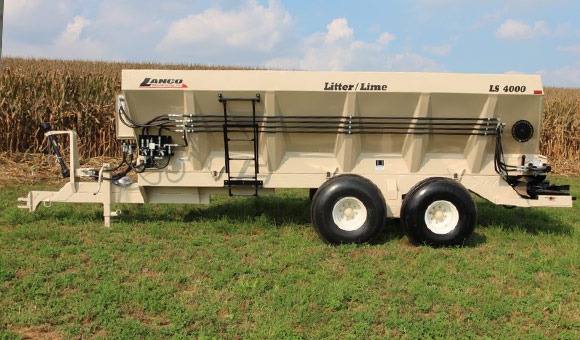The image captures a piece of farm equipment, specifically a trailer branded as "Elanco" with the model name "Litter Slash Lime LS4000". The trailer is off-white or light beige and parked on mowed green grass in front of a late-season cornfield, with the tall, brown plants indicating the time of year. The trailer, which features black hydraulic lines running from the hitch to the back, hints at its function of carrying or distributing some type of material, possibly grain or lime. Prominent on the trailer are large, round black wheels with white hubcaps, and an attached short ladder indicates access to the storage compartment. The sky is a light blue with scattered white clouds, suggesting a clear daytime setting. The trailer, which is not hitched to any vehicle, is viewed from an angle that shows it could be attached to a truck for transport.